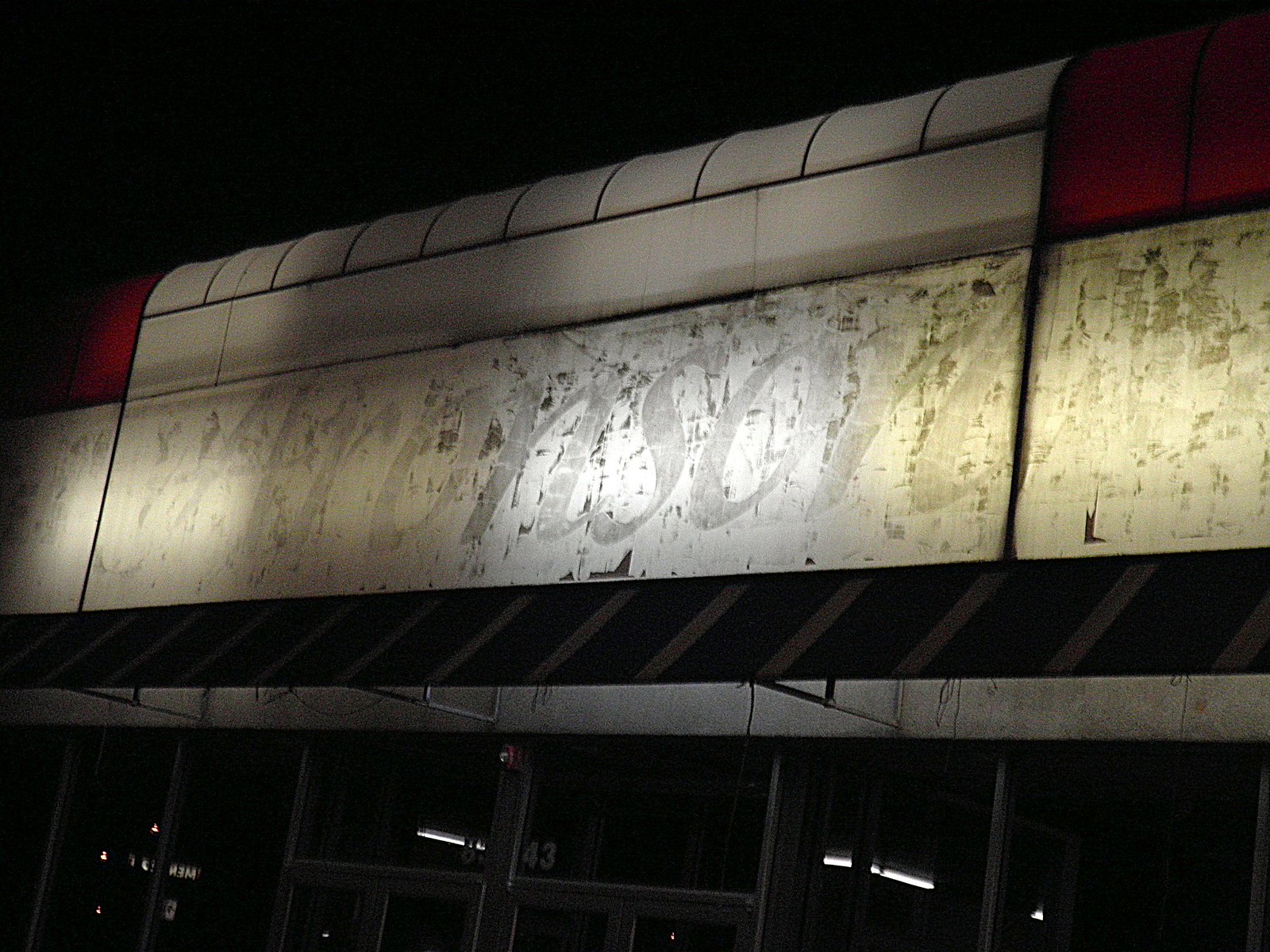The image captures a digital photo taken outdoors at night. The upper portion of the photo is enveloped in complete darkness, presenting a pitch-black sky. Below the sky, the photograph showcases an old, seemingly abandoned store. Situated in the middle of the image, the store has a prominent gray awning that extends upward, oddly arching over the roof.

A weathered sign, originally white with red lettering, hangs from the awning. The sign appears to read "Erickson" in a disjointed cursive style, with each letter separated and heavily faded. The underlying surface of the sign, now looking rusted and brown, hints at its original metallic material.

The store's structure includes black slats forming an open-air roof, connected by a gray strip, and supported by silver columns. Just left of center in the photo, a set of double silver door frames is visible. Above the right-hand door, the number "43" is clearly marked in white.

Additionally, there are intriguing white streaks near the dark windows. These streaks might be reflections of light or perhaps something within the building, adding a mysterious element to the scene.